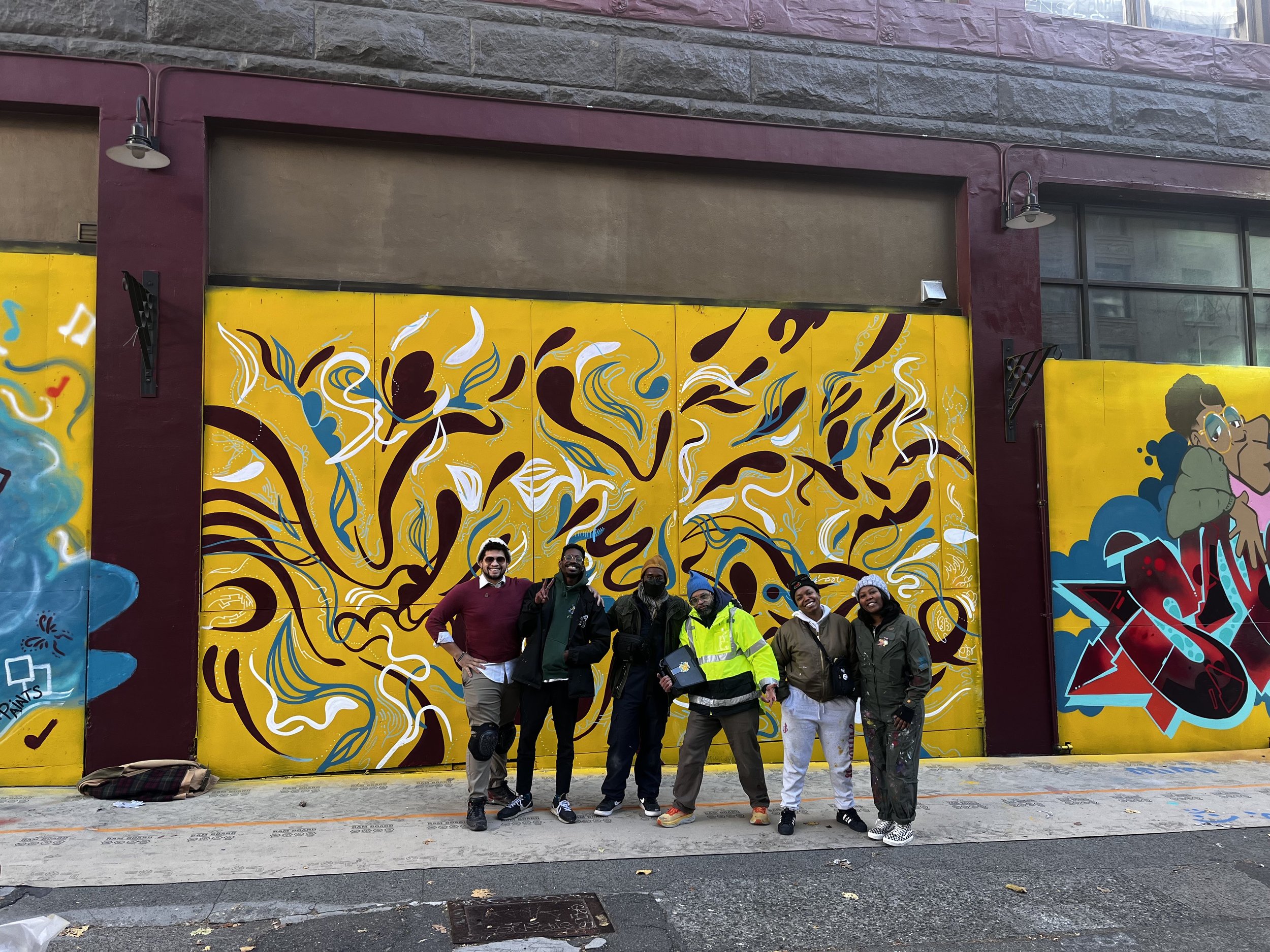This photograph captures a joyful group of six friends standing on an urban sidewalk, which doubles as a construction zone. They are predominantly African-American, with one individual who might be of another race, possibly Mexican or Indian. They are all dressed in construction or painting attire, hinting at their involvement in the creation of the vibrant mural behind them. The backdrop is a graffiti-style artwork on a two-story building's wall, featuring a prominent goldish-yellow background interspersed with abstract designs in maroon, white, and light blue. To the right of the group, there's a striking piece of graffiti art depicting a woman along with some words. The building, possibly an industrial or office space, has a gray stripe above the first floor and is adorned with two lampposts. The friends are all smiling and appear to be sharing a moment of pride and camaraderie, possibly celebrating their artistic contribution to the colorful, professionally executed mural.